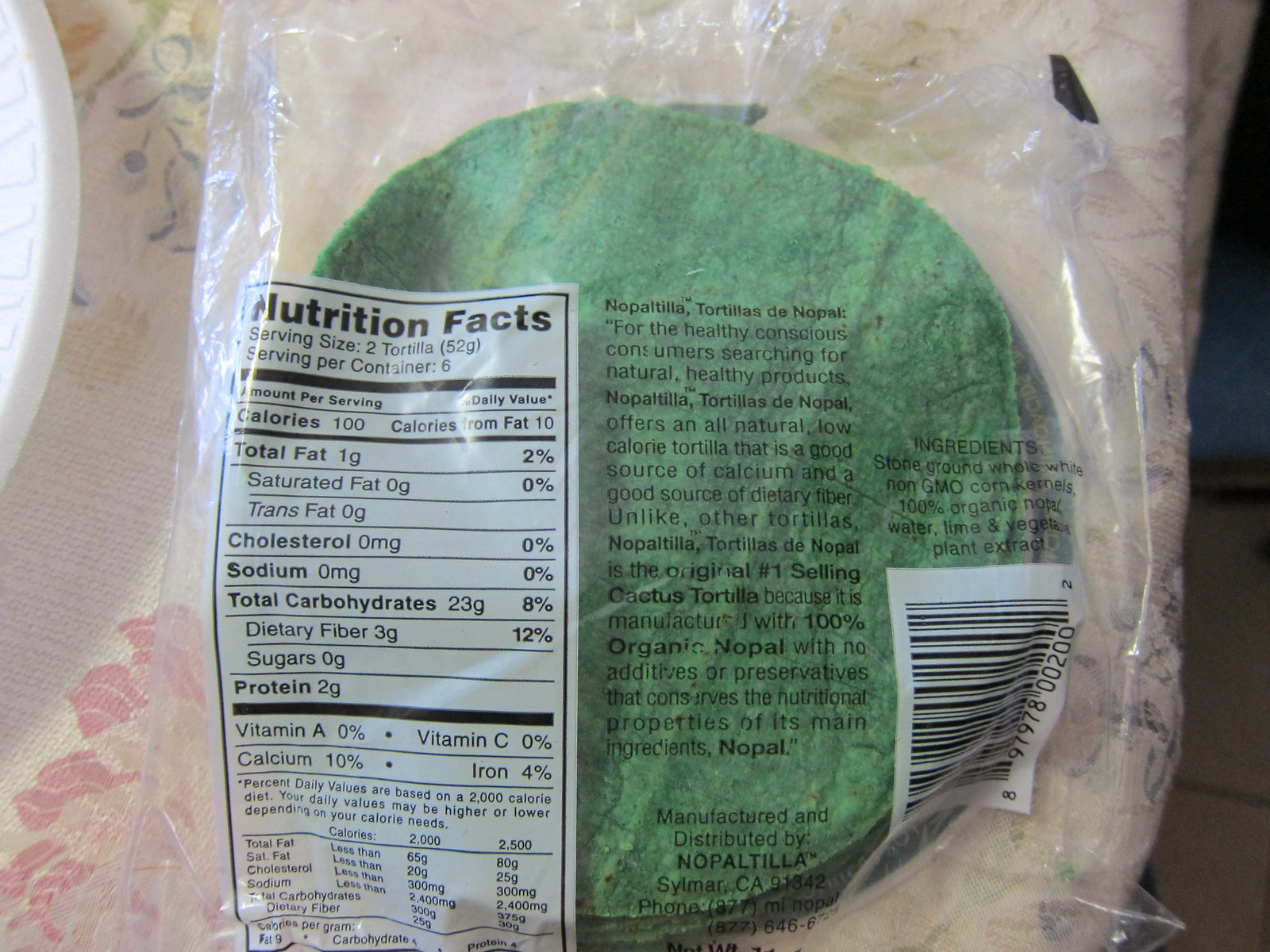The indoor photograph features a table adorned with a white tablecloth decorated with vibrant floral patterns in shades of pink, blue, yellow, and green. Partially visible at the edge of the image is the edge of a plate. Center stage, however, is a clear plastic package containing green tortillas. The back of the package is facing the camera, prominently displaying the nutrition facts and ingredients list. Details reveal that a serving size is two tortillas, with six servings per container, and each serving amounts to 100 calories. Additional elements include a serial number for the ingredients, a barcode, the manufacturer and distributor's name, and a brief product description. The combination of these elements provides a thorough look at the packaged tortillas in a cozy indoor setting.